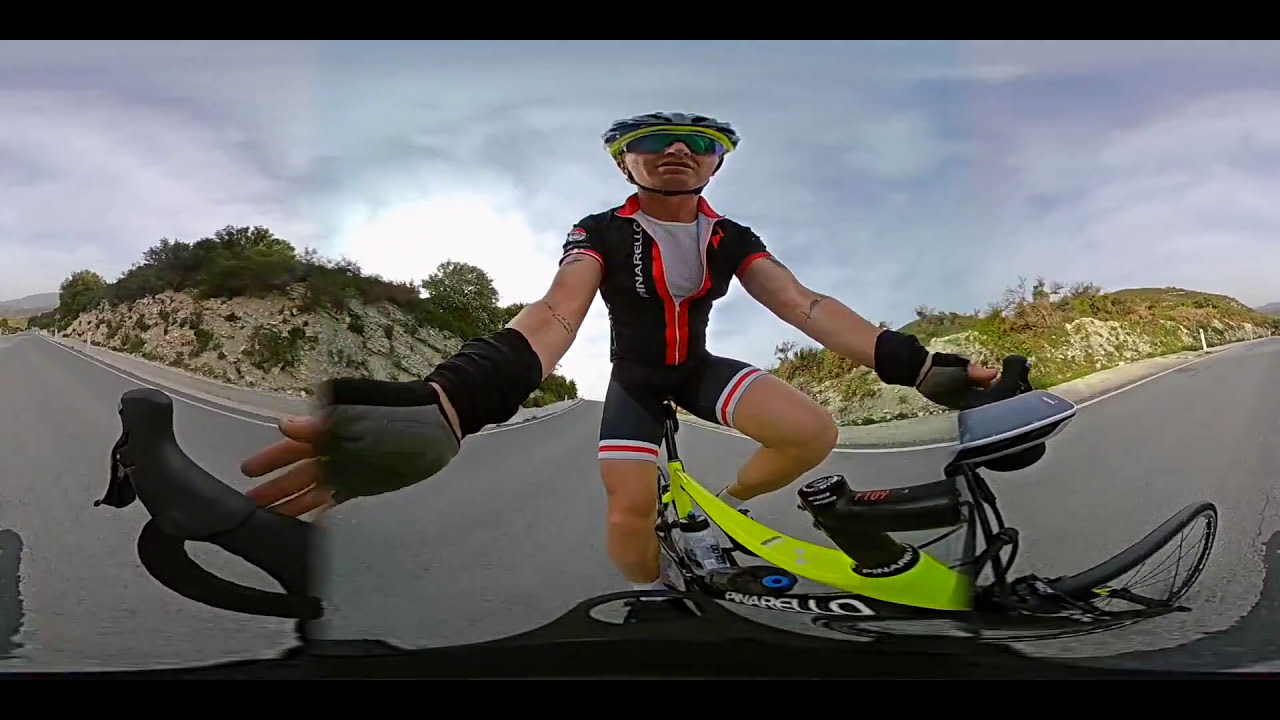The photograph showcases a man riding a professional mountain bike, captured through a wide-angle lens that distorts the image slightly. The biker, presumably in his 20s or 30s, is dressed in a black, short-sleeved, zippered top accented with red, orange, and white details, and matching black biking shorts with similar stripes at the bottom. He wears dark gray or black gloves, a lime green and black helmet, and sunglasses. The bike itself has been variously described as yellow or lime green with black details. The setting features a solitary road with no one else around, flanked by grassy and sandy hills. The terrain appears challenging, with a backdrop that includes rocky sections and scattered plants, all beneath a cloudy sky.